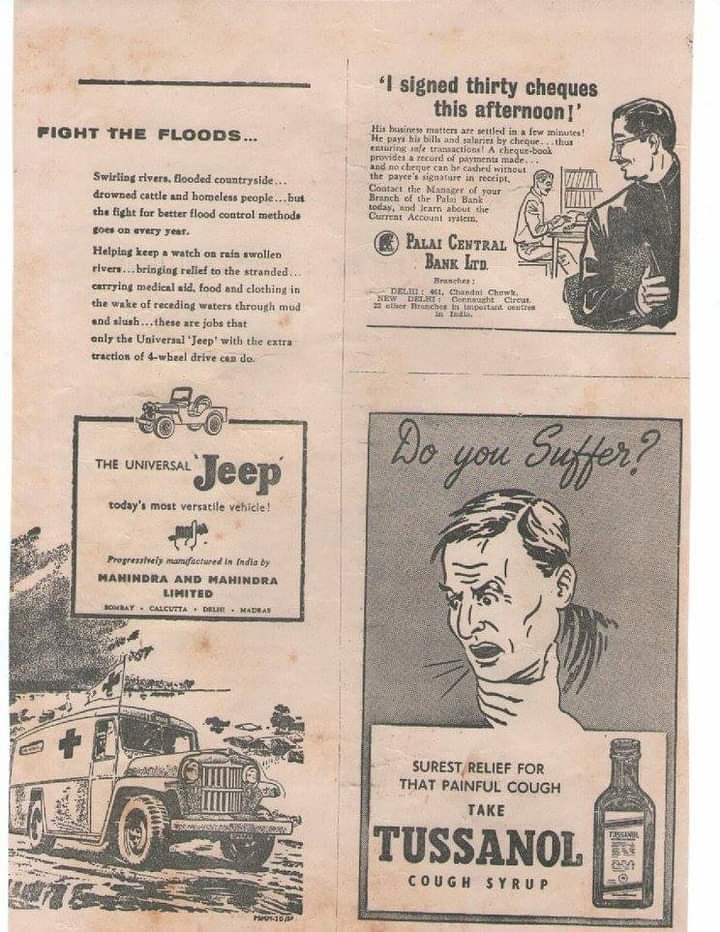This detailed old-time magazine page, likely dating back to the early 1900s, features three black ink-only advertisements, printed on a yellowish-brown, possibly stained surface. The left half of the page is dominated by an ad with the bold headline "Fight the Floods," detailing the relentless struggle against natural disasters. It extols the virtues of the Universal Jeep for its essential role in flood relief efforts, illustrating a classic jeep and an emergency medical vehicle. The text beneath underscores the jeep's versatility and reliable four-wheel drive, noting its manufacture by Mahindra and Mahindra Limited in India.

In the top right corner, another advertisement states, "I signed 30 checks this afternoon," promoting Palai Central Bank Limited. It features an illustration of two men, one exiting an office while the other remains at a desk, hinting at the ease and efficiency of their banking services.

The bottom right corner presents an ad with a grey background, headlined "Do you suffer?" in cursive. It includes the illustration of a man coughing, advocating for Tuscanol Cough Syrup as the surest relief for painful coughs. Each segment offers a glimpse into the products and services of the era, unified by their practical appeals and illustrative storytelling.